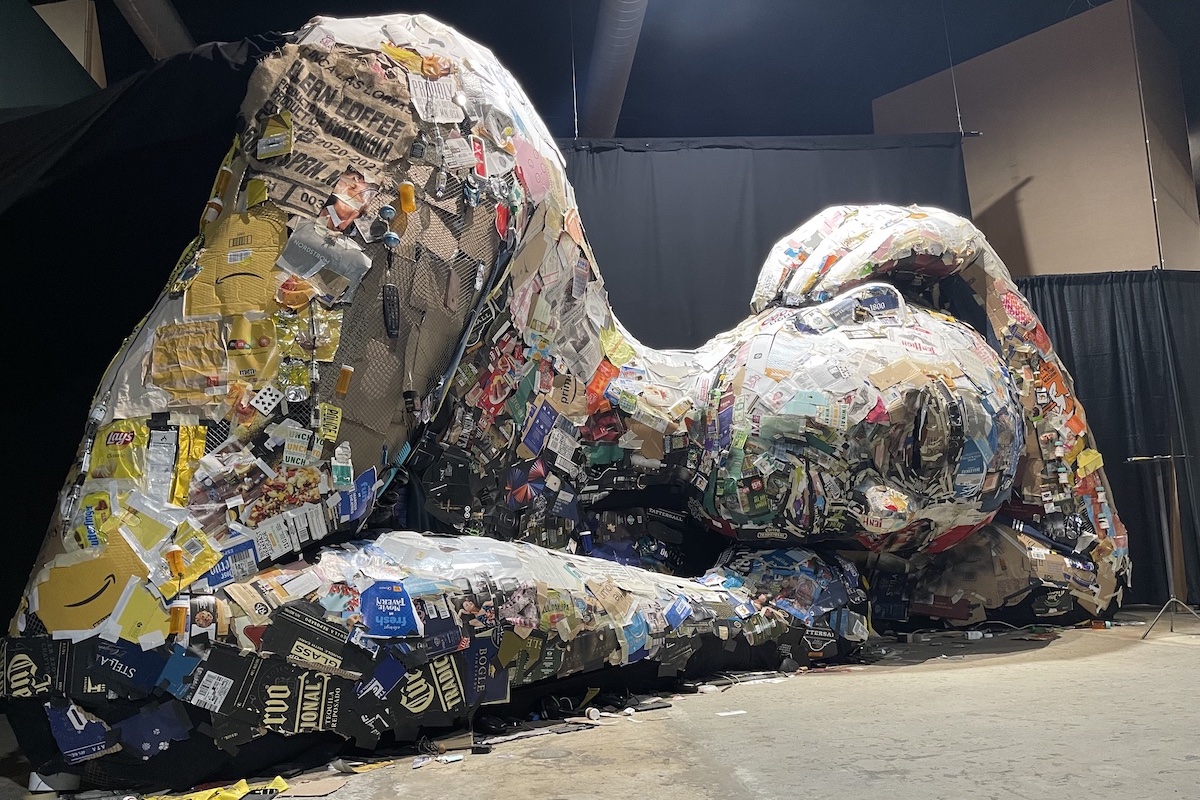The image depicts a large, gray human-shaped sculpture displayed in an art studio. The figure, assembled using various pieces of paper mache, is lying on its side with its head resting on what appears to be an arm or a pillow. One hand is placed over its ear, emphasizing a sense of repose. The sculpture is adorned with a mosaic of paper, including labels and fragments from everyday items like Amazon boxes and possibly a Corona label, in a variety of colors such as yellow, blue, and black. The background features both tall and shorter black curtains, and the floor is concrete, framing the detailed and textured surface of the artwork.